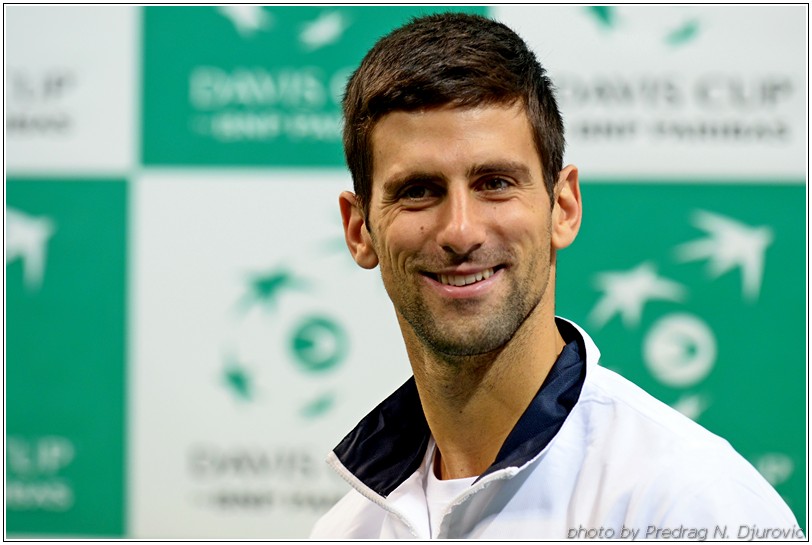This image captures tennis star Novak Djokovic standing at the center, smiling directly at the camera. He is a Caucasian man with short, clean-cut brown hair and the beginnings of a brown beard and mustache. His smile reveals a glimpse of his front teeth. He is dressed in a mostly zipped-up white jacket with a dark blue collar lining and a white undershirt visible underneath. The background is somewhat blurred, revealing a green and white checkered pattern with indistinct logos that appear to be green birds, stars, and circular shapes against alternating mint green and white squares. A watermark at the bottom right corner reads "Photo by Predrag N. Djokovic" in blackish-gray text. The setting suggests an indoor or outdoor sporting event.